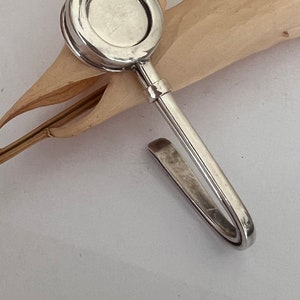The image displays a detailed scene of two distinct objects resting on a light gray surface. At the forefront is a cylindrical wooden object with a carved, almost triangular cut near its end that resembles an open mouth or flower petal shape. Emerging from this triangular opening is a narrow rectangular wooden rod. Positioned atop this wooden piece is a silver object that closely resembles an antique stopwatch. The silver instrument features a circular head with a blank, white inlay, akin to a watch face without numbers. Extending from the head is a metal tube that curves downward, forming a flat stem on which the silver piece rests. The entire scene is subtly shadowed to the lower left, adding depth to the intricate composition. Both objects are partially visible, with the silver piece slightly cut off at the top, creating a well-balanced and intriguing visual.